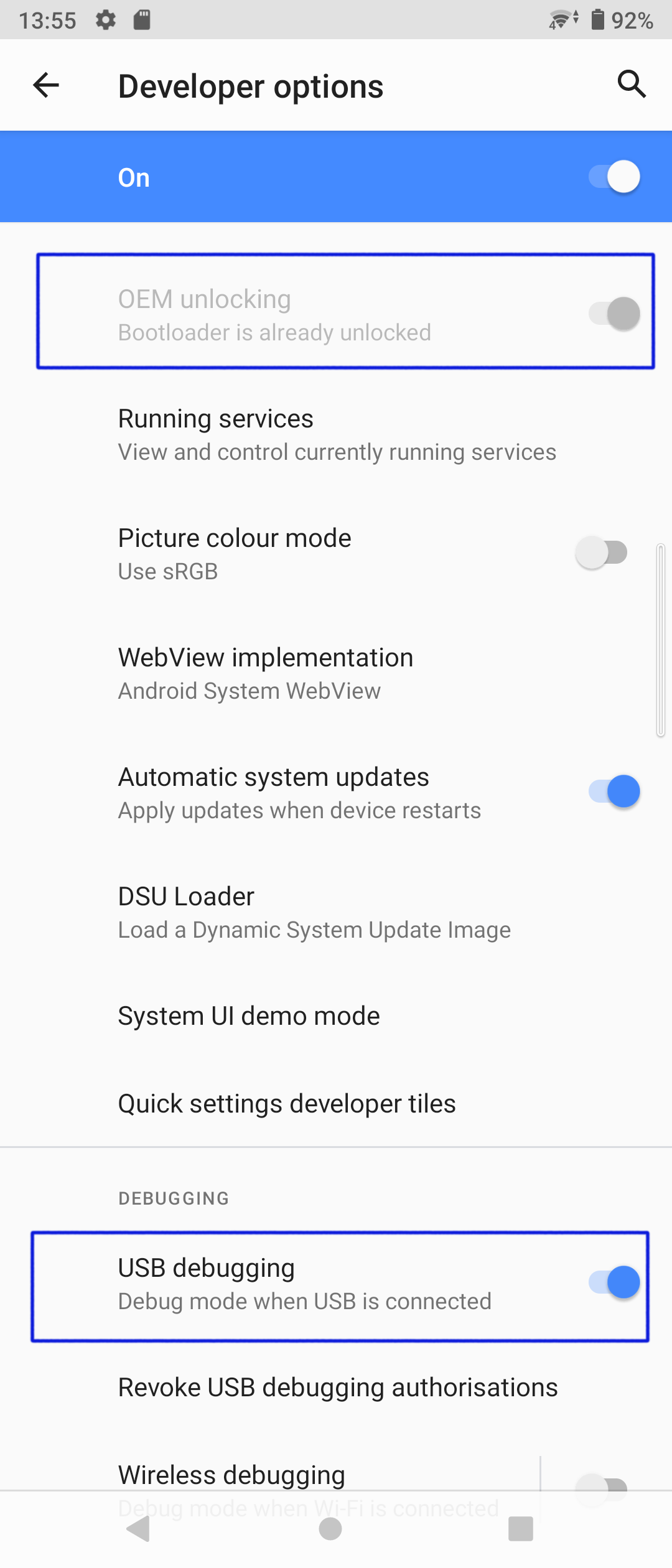Screenshot of Developer Options Menu

The image is a screenshot of an Android device's Developer Options menu. Set against a white background, there is a light gray header at the top. In the header, the time "13:55" is displayed in black text on the left side. The right side of the header contains a black settings icon, a Wi-Fi signal icon, and a battery icon indicating a 92% charge.

Beneath the header, the main content area features the title "Developer options" in black text on a white background. Below this title, a blue button is labeled "On" with a toggle switch turned to the right, indicating that Developer Options are enabled.

The following options are listed below the main title:
1. OEM unlocking - Light gray text with the description "Bootloader is already unlocked," enclosed within a blue border.
2. Running services - Described as "View and control currently running services."
3. Automatic system updates - Accompanied by a toggle switch on the right, which is turned on.
4. DSU loader - Described as "Load a dynamic system update image."